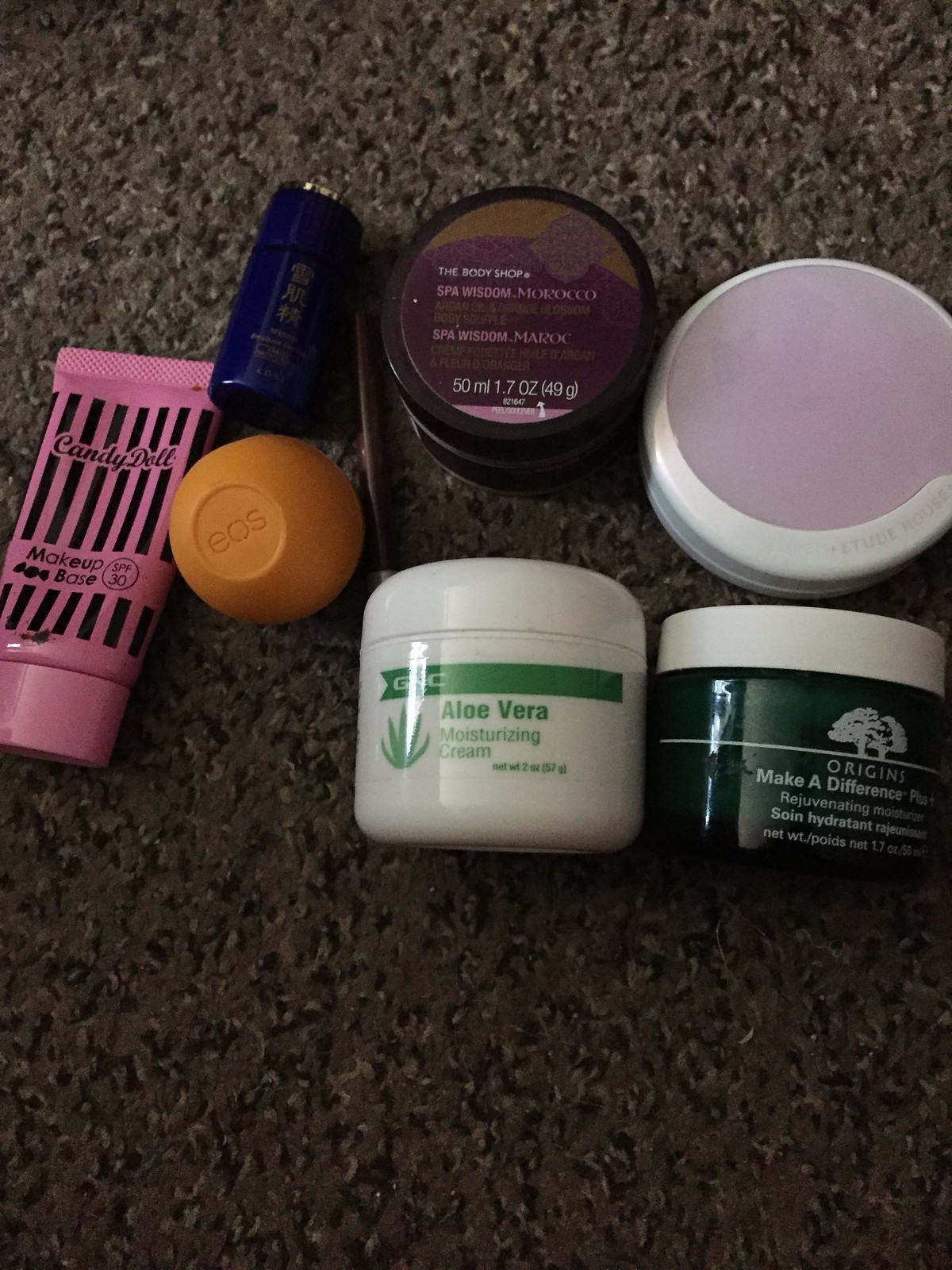In the image, a variety of skincare and makeup containers are meticulously arranged on a dark brown low-pile carpet, creating an organized yet casual display of personal grooming products. There are seven distinct items, each with specific features and branding.

Starting from the right:

1. **Candy Doll Makeup Base**: A pink and black striped squeeze tube with SPF 30, adorned with black lettering. It features a convenient flip cap on the bottom.
  
2. **EOS Lip Balm**: Encased in a cheerful yellow-orange spherical container, easily recognizable with the “EOS” logo engraved on its flat top.
  
3. **Asian Product**: Positioned above the lip balm, this small dark blue item has writing in either Chinese or Japanese, making it difficult to identify the exact product type.
  
4. **Eyebrow Pencil**: Nestled next to the EOS lip balm and the Asian product, hinting at its role in precise makeup application.
  
5. **The Body Shop Spa Wisdom Morocco**: Located on the top row, this round container features a screw-off top and is emblazoned with the “Spa Wisdom Morocco” label. Although its exact function is unclear, it might be a body scrub or a similar product. It holds 50 milliliters (1.7 ounces).
  
6. **GNC Aloe Vera Moisturizing Cream**: Below the Body Shop product, this white cylindrical container with a screw-off top features green lettering and an aloe plant image, indicating its soothing aloe vera content.
  
7. **Unidentified Cylindrical Container**: On the top row again, another mysterious white cylindrical container with a light purple top, devoid of identifying marks or labels.
  
8. **Origins Make A Difference Rejuvenating Moisturizer**: Completing the arrangement, this dark green cylindrical container with a white screw-off top is embellished with tree illustrations above a white line. The branding clearly states “Origins” and “Make A Difference,” followed by “rejuvenating moisturizer” in both English and French.

This ensemble of products highlights a comprehensive range of grooming essentials strategically organized on a carpet, showcasing both known brands and enigmatic items.